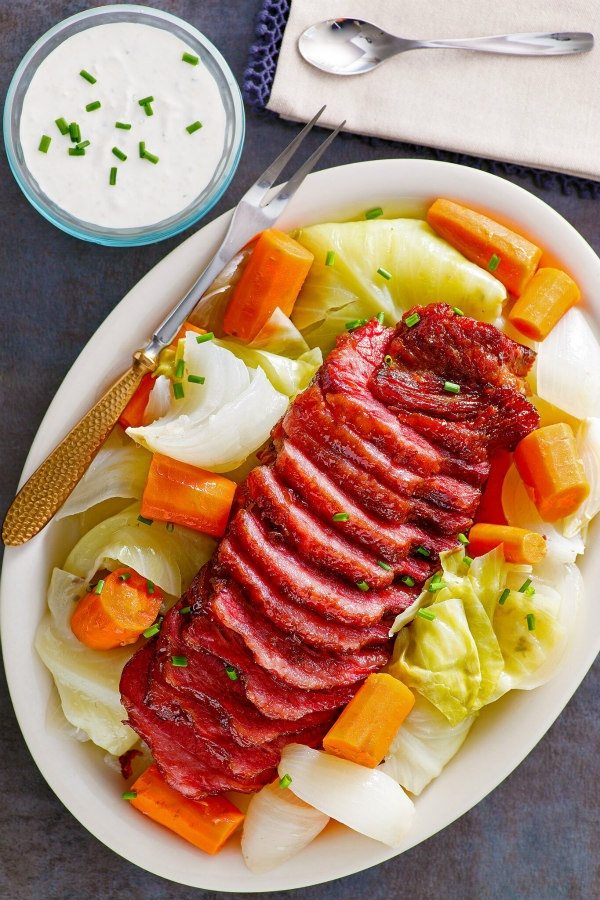The image depicts an overhead, bird's-eye view of a meticulously arranged meal set on a dark gray, purple-hued table. Central to the composition is a large, cream-colored oval plate positioned diagonally. On the plate is an enticing dish featuring evenly sliced, vibrantly colored red roast beef, surrounded by assorted vegetables including large, bright orange carrots and light green boiled cabbage. Additional green chives are scattered atop the beef for a pop of color. To the top left of the plate, a glass bowl filled with white sour cream garnished with 16 meticulously placed chives adds a decorative touch. The top right-hand corner features a cream-colored napkin with a purple embroidered trim, neatly folded beneath a silver spoon extending into the center of the image. The peripheral areas of the image display the dark gray table background, emphasizing the vibrancy and arrangement of the meal. The detailed, restaurant-quality presentation draws the viewer's eye to the carefully crafted culinary display.